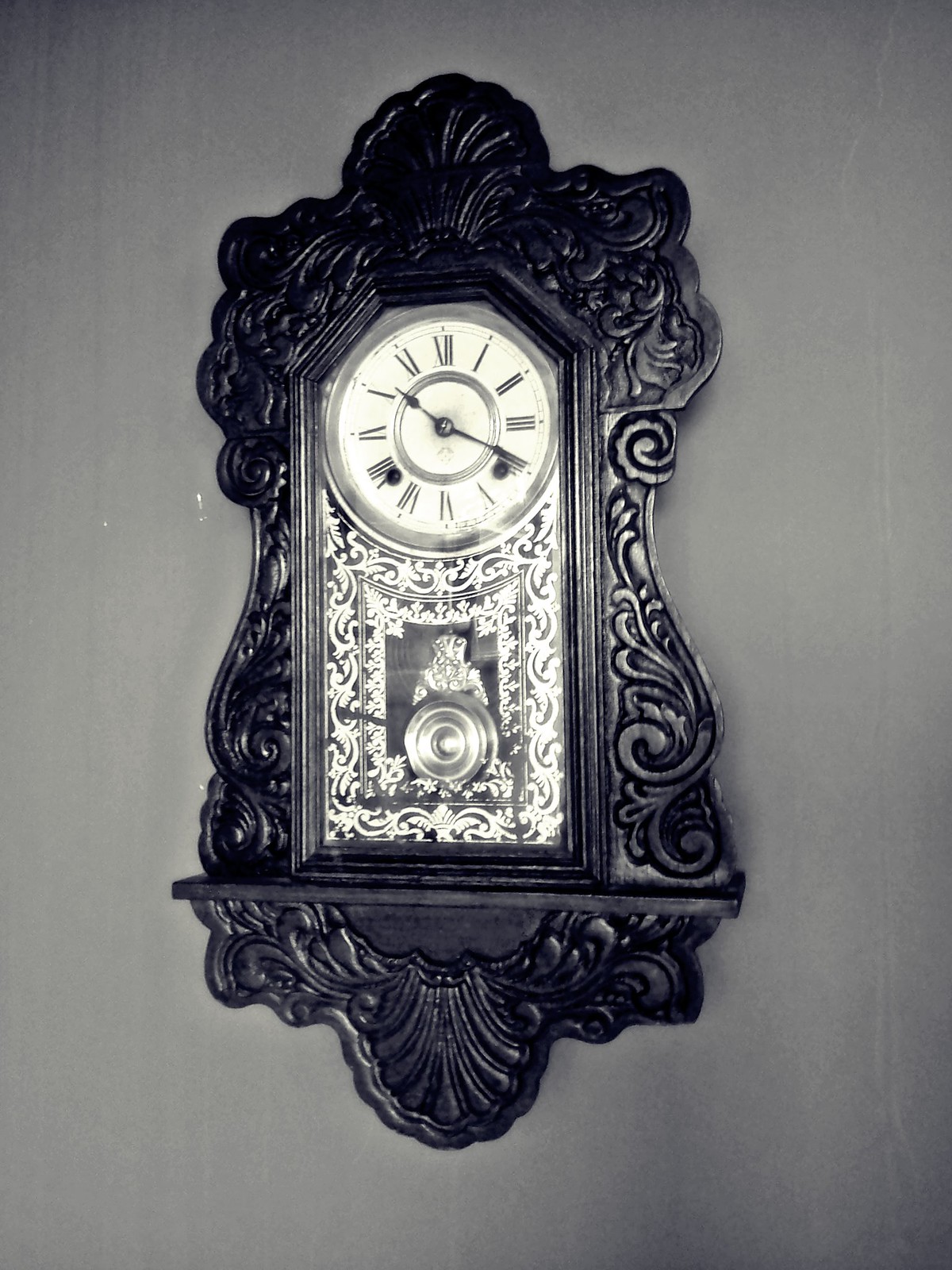This black-and-white photograph showcases an exquisitely ornate clock mounted on a wall. The clock features a distinctive oblong, rounded square shape, adorned with intricate seashell motifs at both the top and bottom, adding a touch of elegance to its design. The dark-colored frame encases an inner metal inlay embellished with detailed patterns. Prominently displayed within this frame is a swinging pendulum, hinting at the clock's mechanical nature. The clock face itself stands out with Roman numerals instead of traditional numbers, further enhancing its classic appeal. The time indicated on the clock is approximately 10:20. The monochromatic nature of the image emphasizes the timeless beauty of the clock's craftsmanship without the distraction of color.